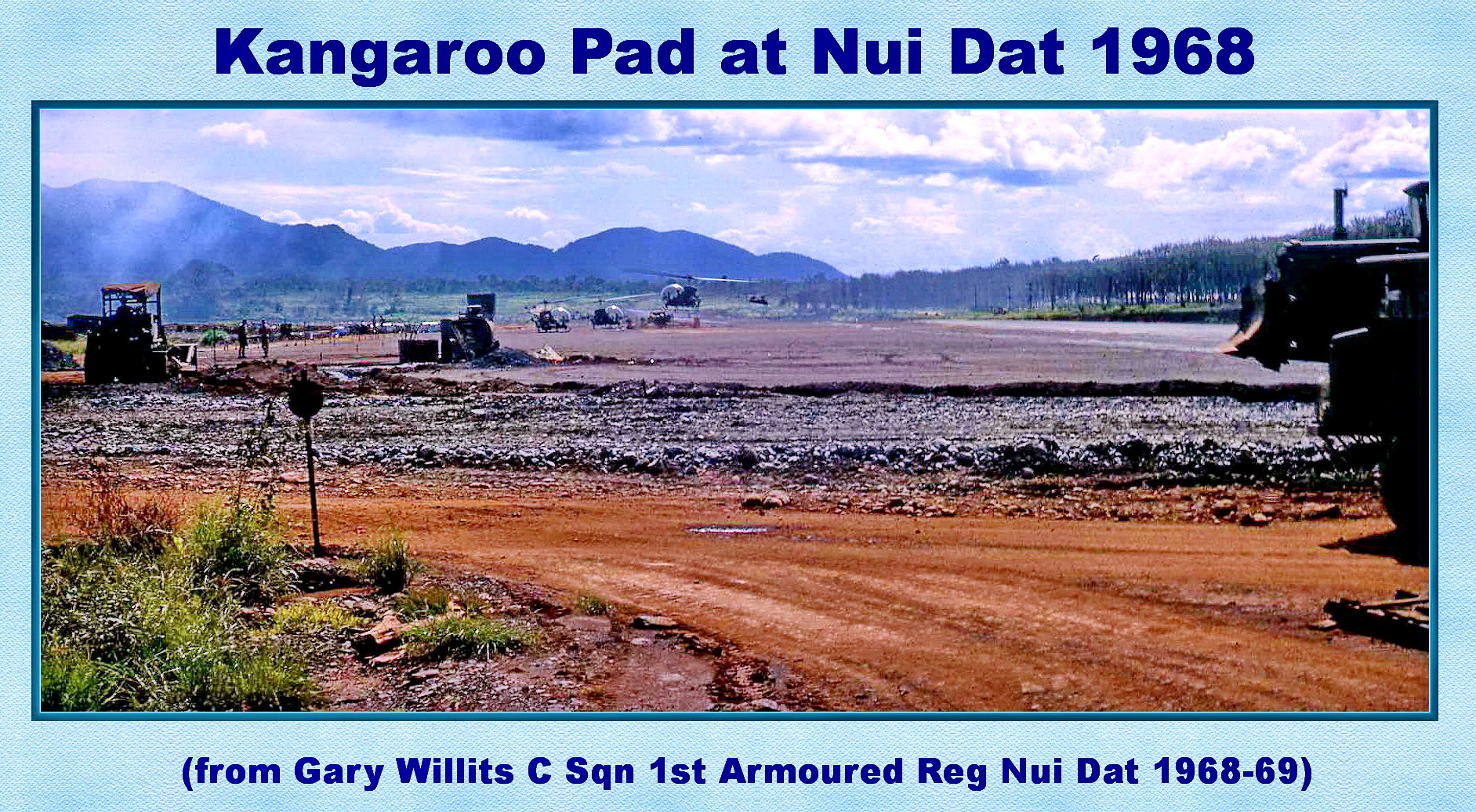A vintage photograph titled "Kangaroo Pad at Nui Dat 1968" with the caption "From Gary Willetts, C. Squan First Armored Regiment, Nui Dat 1968-69" at the bottom features a dirt road leading from the left and splitting to the right. In the foreground, the road transitions to a gravel path on the right, with a signpost on the left, partially obscured. The landscape is reminiscent of a war zone in Vietnam. Two small helicopters are visible, one just off the ground and the other stationed on the ground. Heavy machinery, possibly a bulldozer or tractor, is positioned on the left. Green weeds and patches of dirt are evident in the bottom left corner. The background reveals an orchard of trees on the right, and the silhouette of blue mountains across the horizon, which diminish in height from left to right until they disappear near the center. The sky showcases a mix of blue with white cloud coverage, capturing the rural and somewhat barren scenery of Nui Dat during 1968.